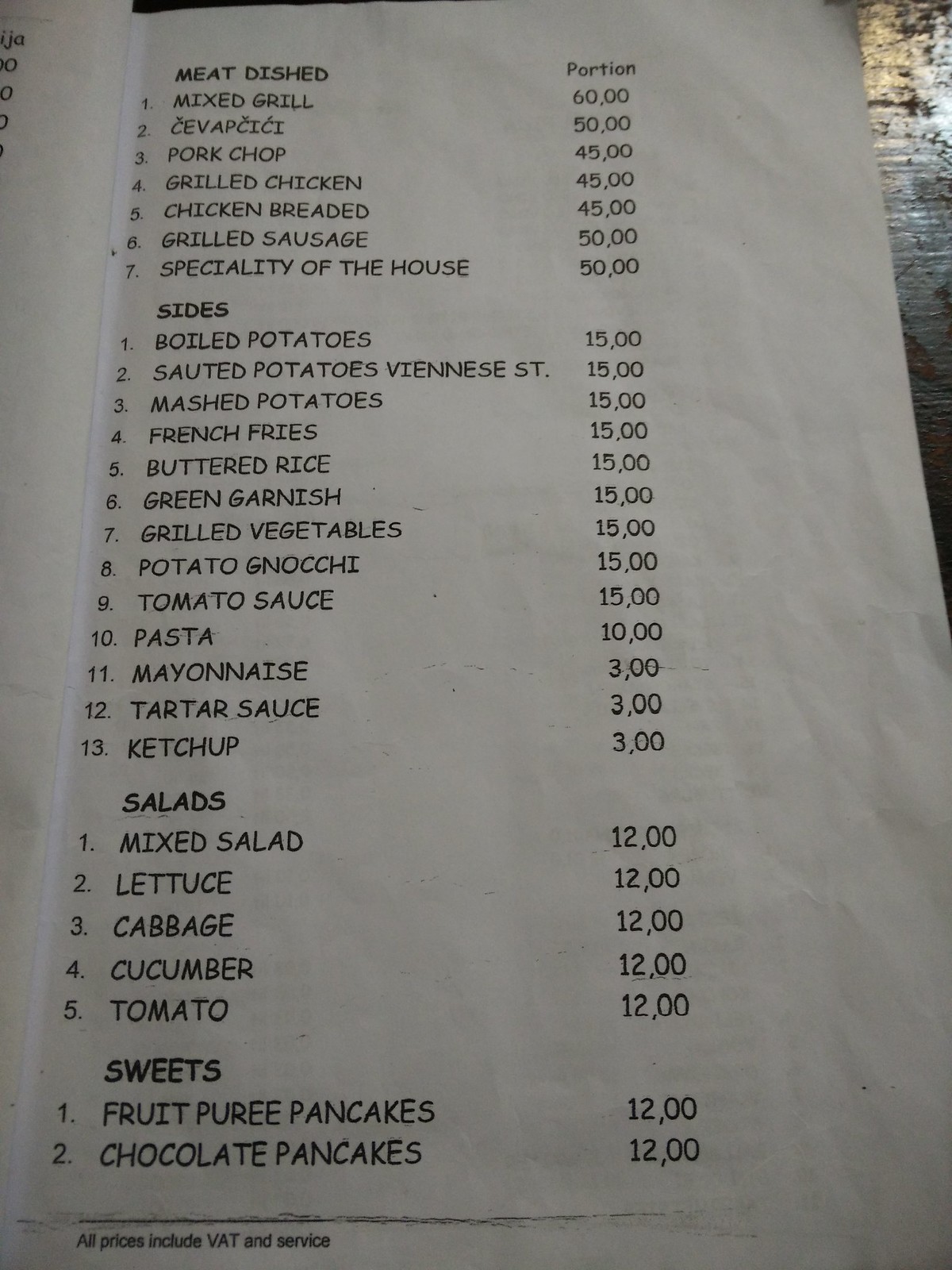This photo captures a detailed view of a food menu printed on regular white paper and bound in an open booklet format. The menu is meticulously organized by categories, each with numbered items and corresponding prices. On the left page, the "Meat Dishes" section lists seven options: mixed grill, pork chops, grilled chicken, chicken breast, and grilled sausage, along with a house specialty, all priced between $45 and $60. The sides category features 13 items, including various types of potatoes, condiments, and vegetables. Salads, numbered one through five, include options like cabbage, cucumber, and tomato. The sweets section, simple yet enticing, offers two types of pancakes. Each dish's name and its cost or portion size are neatly displayed, ensuring clarity and ease of selection for patrons.